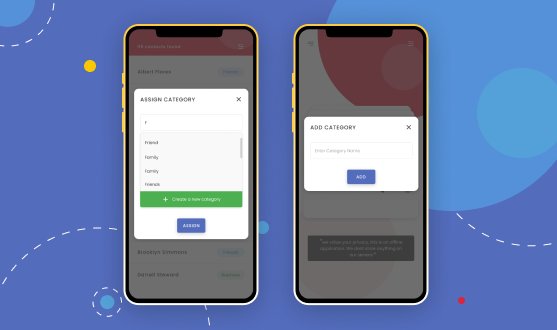The image features a rectangular blue box with a visually engaging background comprised of circles and dotted line circles. To the left, there are several yellow circles adding a vibrant contrast to the various shades of blue. Centrally positioned within this blue box are two iPhone mockups. 

The left iPhone screen displays an interface with options labeled "Assign Category." Below this label, the options include "Friend," "Family," "Family Friend," and "Create Category." The right iPhone mockup shows a screen with the option "Add Category," suggesting the user can create custom categories. The app interface presented on the iPhones has a red background, providing a stark contrast to the blue-themed environment of the overall image.

This mockup appears to be part of a presentation potentially illustrating how to use the app, which could be for organizing contacts or managing finances based on the categorization feature.